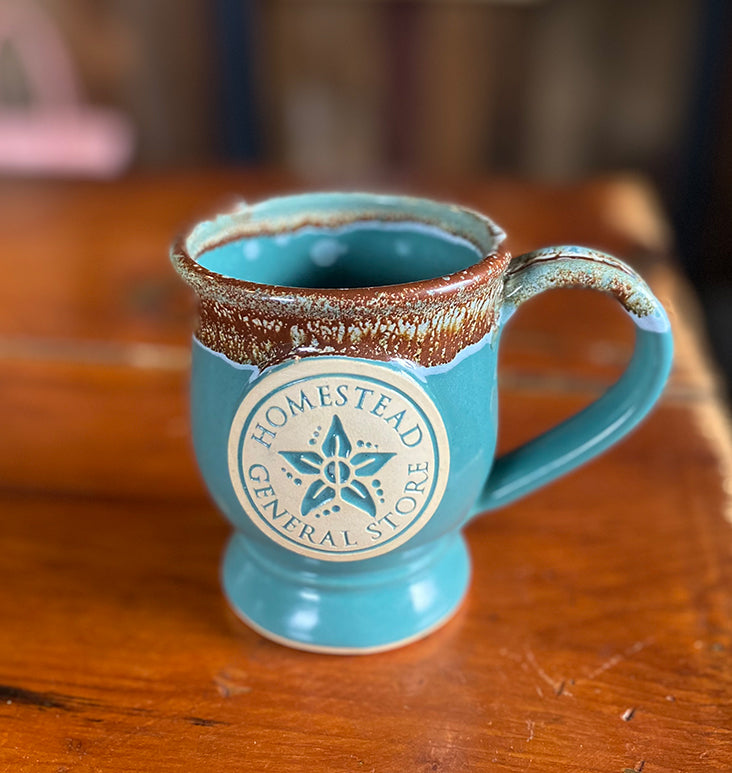The image features a rustic, weathered mug from the Homestead General Store. The mug’s design is primarily bright blue with a weathered brown trim near the top, which fades and reveals more blue speckles due to the worn glaze. "Homestead General Store" is carved into a white circular area bordered in blue, with a flower logo consisting of a circle and five petals intersected by lines right at the center. The large handle on the right is shaped like half of a heart, with the top section exhibiting the same brown and weathered appearance as the rim. The mug is empty and stands on a worn, orange-brown wooden table, while the background is artistically blurred. The photo captures the mug in a detailed, portrait-like style, enhancing its vintage charm.